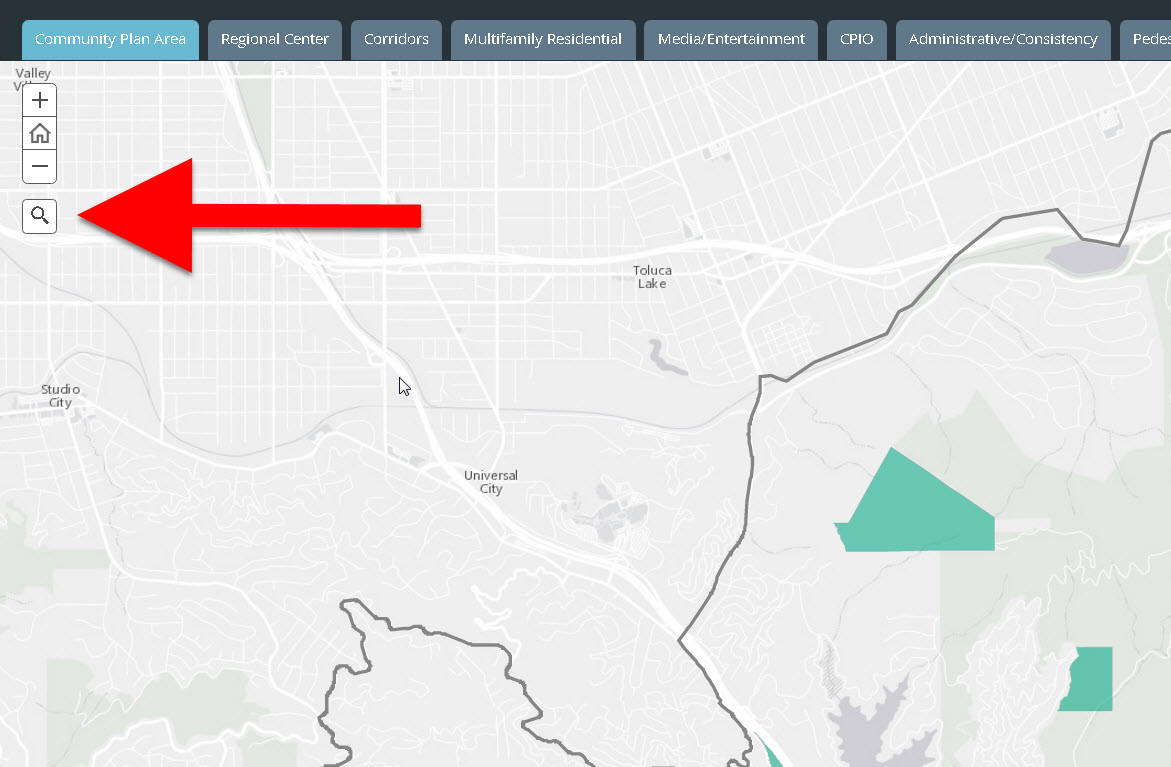This image depicts a GPS navigation interface or a topographical map designed for governmental or administrative use. At the top left corner, a series of tabs are displayed in a medium gray color with white text. The currently selected tab is "Community Plan Area," while the other available tabs include "Regional Center," "Corridors," "Multifamily Residential," "Media/Entertainment," "C-P-I-O," "Administrative/Consistency," and a seemingly truncated tab starting with "Pedest...," likely referring to "Pedestrian."

The map features various streets, possibly lakes, and trails, providing a detailed view of the area's geography. The cities labeled from left to right on the map are Studio City, Universal City, and Toluca Lake. A noticeable red arrow points to the left towards a search icon, suggesting that this image might be serving as an instructional guide on how to navigate or utilize the interface.

Overall, this detailed cartographic representation illustrates how different zones within the specified cities are organized and highlights essential navigational tools within the system for effective usage by professionals.